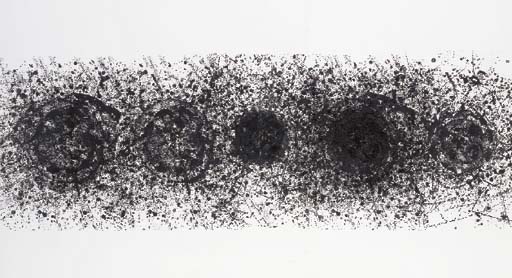The image is a horizontally aligned, rectangular artwork set against a light gray background. It features a rectangular pattern of finely dispersed black dots, which become denser toward the middle. Centered within this pattern are five circular shapes arranged in a linear sequence. From left to right, the first and second circles have a spiral design, with the second showing more intricate details. The middle circle is the smallest and almost completely blackened. The fourth circle is similar in density to the middle one but larger, with faint swirls surrounding its nearly filled black interior. The fifth and final circle, on the far right, also features a spiraled pattern. Collectively, these circles and the dot pattern evoke an artistic representation reminiscent of atomic structures, with dynamic, indeterminate movements akin to electrons around an atom.